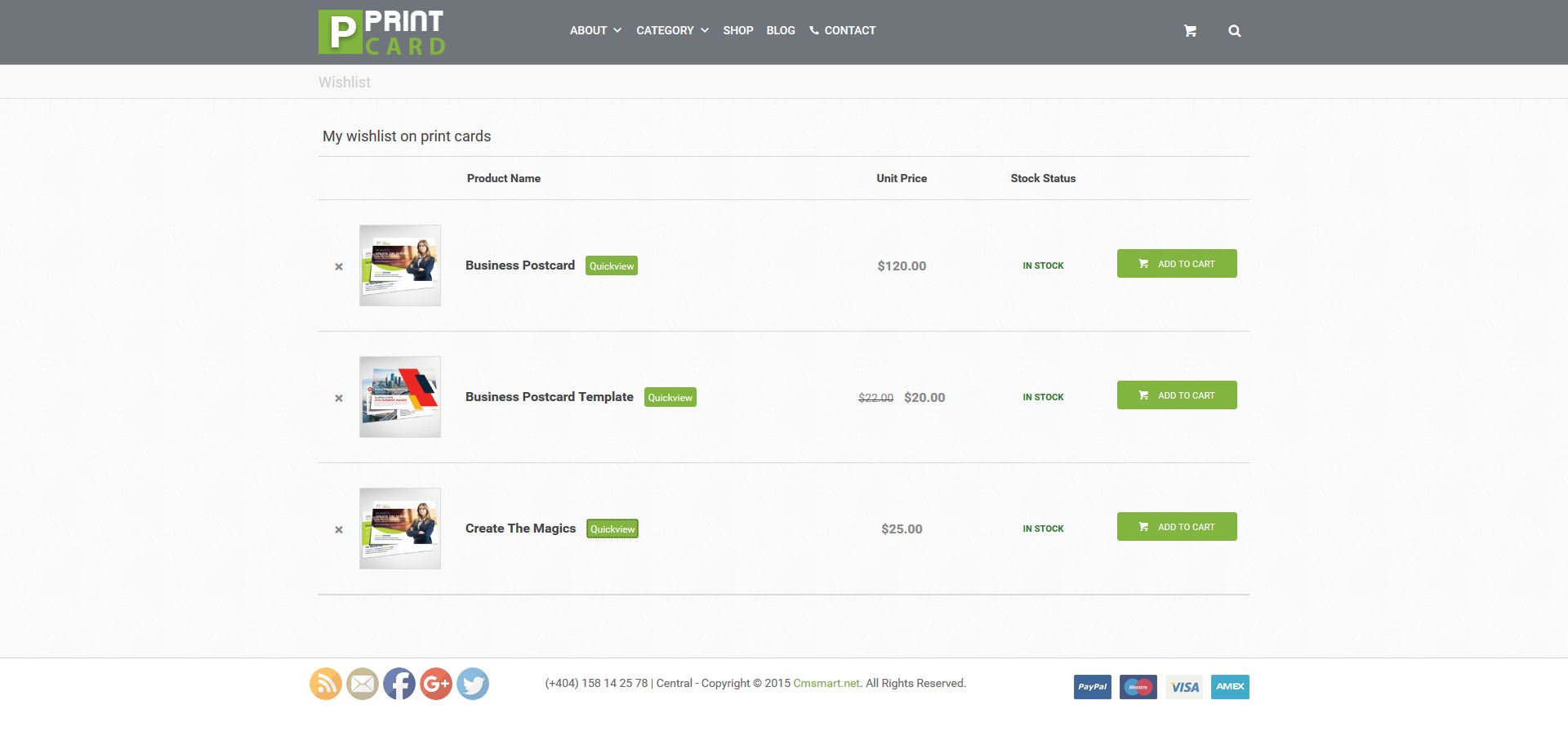Here is a clean and detailed caption for the image described:

---

The website features a clean and organized layout for "Print Card." At the top, there's a gray navigation bar with a prominent green square containing a white, uppercase "P" signifying the Print Card logo. The navigation menu includes options such as "About" with a drop-down menu, "Category" with another drop-down, "Shop," "Blog," and a "Contact" link marked by a phone icon. To the far right, the bar hosts a shopping cart icon and a search magnifying glass icon.

Below the navigation bar, a light gray line holds the "Wish List" link, leading to a page titled "My Wish List on Print Card." This page features several products listed in a column.

1. **Business Postcard**: 
   - **Icon**: Green "X"
   - **Image**: Woman standing with a box
   - **Product Label**: Business Postcard
   - **Button**: Green "Quick Home" button
   - **Unit Price**: $120
   - **Stock Status**: In stock (green text)
   - **Cart Button**: Green add to cart button with a white shopping cart icon and white text

2. **Business Postcard Template**: 
   - **Icon**: Green "X"
   - **Image**: Papers and business cards
   - **Product Label**: Business Postcard Template
   - **Button**: Green "Quick Home" button
   - **Original Price**: $22 (crossed out)
   - **Sale Price**: $20
   - **Stock Status**: In stock (green text)
   - **Cart Button**: Green add to cart button with a white shopping cart icon and white text

3. **Create the Magics**: 
   - **Icon**: Green "X"
   - **Image**: Same woman as in Business Postcard
   - **Product Label**: Create the Magics
   - **Button**: Green "Quick Home" button
   - **Unit Price**: $25
   - **Stock Status**: In stock (green text)
   - **Cart Button**: Green add to cart button with a white shopping cart icon and white text

At the bottom of the website are various social media icons, a customer service phone number (404-158-142578), and copyright information. The footer reads "© 2015. All rights reserved." with an almost unreadable URL (possibly c-mart.net). Additionally, logos for payment methods, including PayPal, MasterCard, Visa, and American Express, are prominently displayed.

---